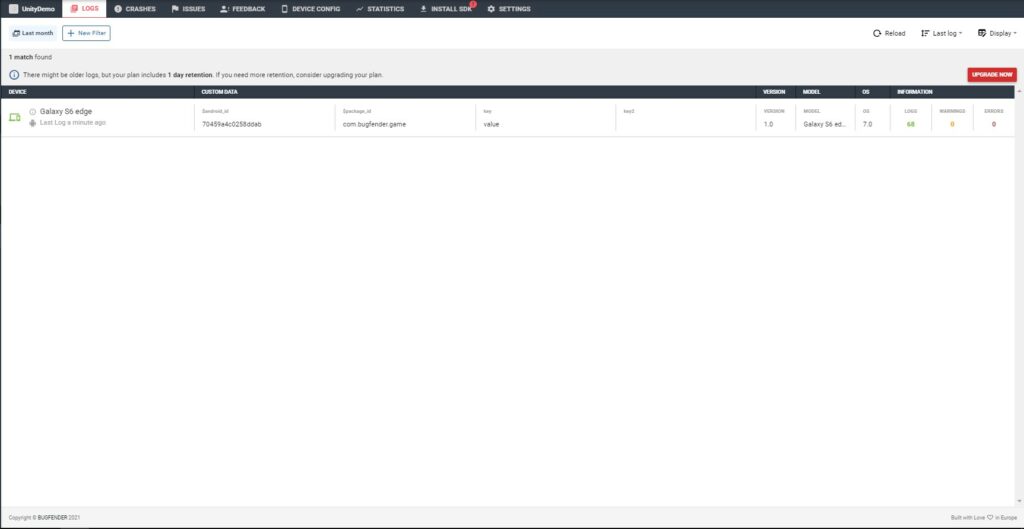The image depicts a blurred screen capture of a web page displayed on a desktop computer. The page features a subdued background with varying shades of grey and a faint pastel hue. Prominently, in the upper right corner stands out a red rectangular button, offering contrast amidst the otherwise muted tones. The top section of the page is characterized by two black horizontal bars. The uppermost bar houses several menu options, clearly evident due to the white font against the black background. Below a brief expanse of empty white space, a second black horizontal bar mirrors the first, also containing more menu options in white text. Following this bar, the page displays multiple lines of data entries; however, the text is so blurry and faint that the specific details are indiscernible. The remainder of the web page below these entries is devoid of content, appearing blank.